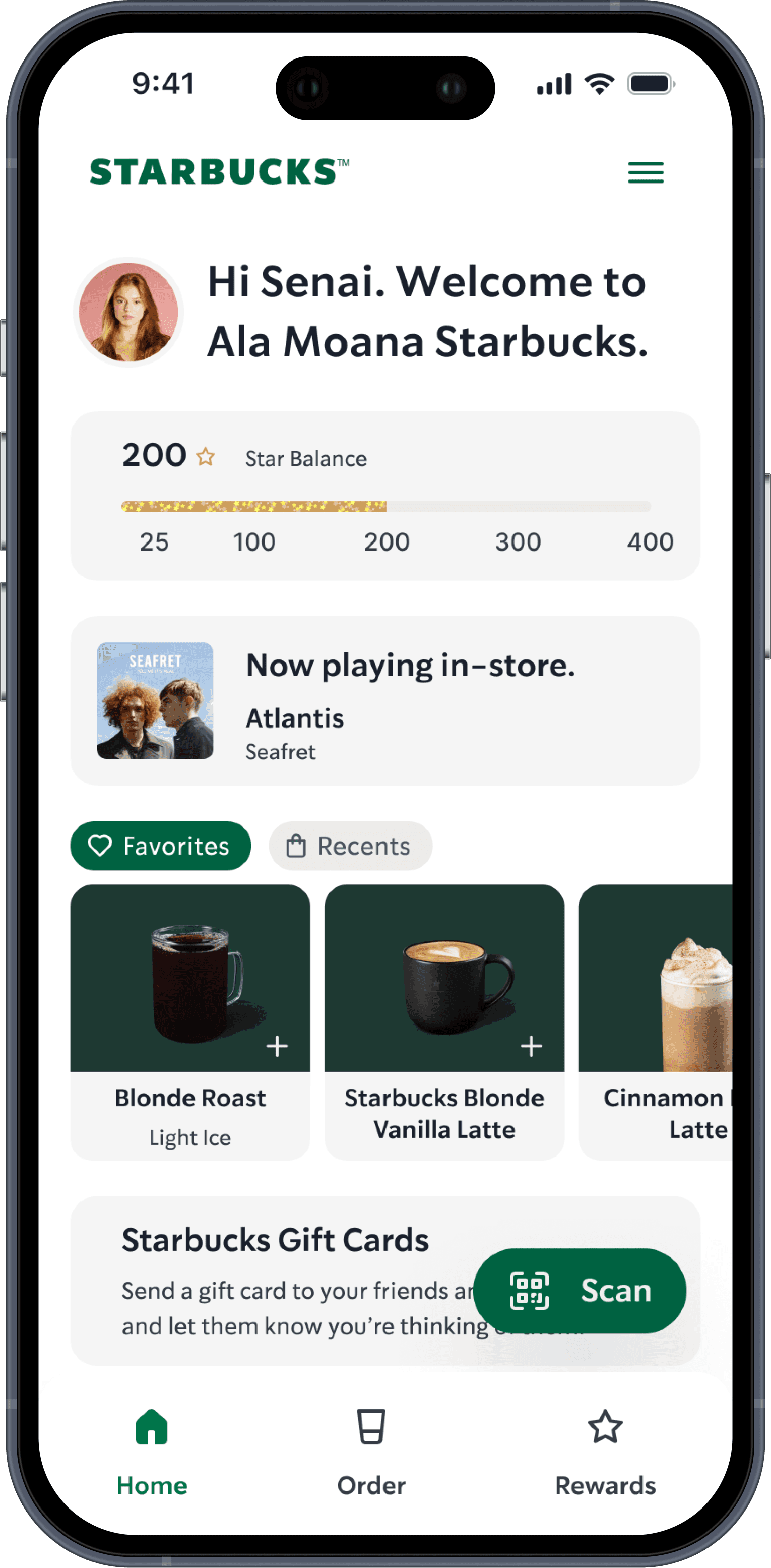In this detailed mock-up, an individual is holding an iPhone displaying the Starbucks app. The phone's outer metal band and buttons are clearly visible. On the top-left corner of the screen, the time reads 9:41. The status indicators show four bars of signal, full Wi-Fi connectivity, and a fully charged battery. 

The Starbucks app interface features a clean white background. Prominently positioned is the classic green Starbucks logo, albeit without the iconic mermaid. To the right, three bars form a hamburger menu. Adjacent to this, there is a circular profile picture of a woman. The app greets the user with "Hi, Sene (S-E-N-E-I). Welcome to Ala Moana Starbucks."

The star balance, prominently displayed, currently stands at 200, aligned with markers for 25, 100, 200, 300, and 400 stars. Below this, there's a notification area indicating "Now playing in store: Atlantis by Seafret," hinting at the app's multimedia capabilities.

Further down, options labeled "Favorites" and "Recent" in green pill-shaped buttons are visible. Under "Favorites," drinks such as Blonde Roast with light ice, Starbucks Blonde Vanilla Latte, and a partially visible Cinnamon Latte are listed, each accompanied by pictures on dark green backgrounds.

A section offering Starbucks gift cards tells users to "Send the gift cards to your friend and let them know you're thinking of them," though the text is partially obscured by a green, capsule-shaped button with a QR code icon and the word "scan" next to it.

At the bottom of the app screen, there are navigation icons: a green house labeled "Home," a gray coffee cup with "Order" beneath it, and a "Stars and Rewards" section.